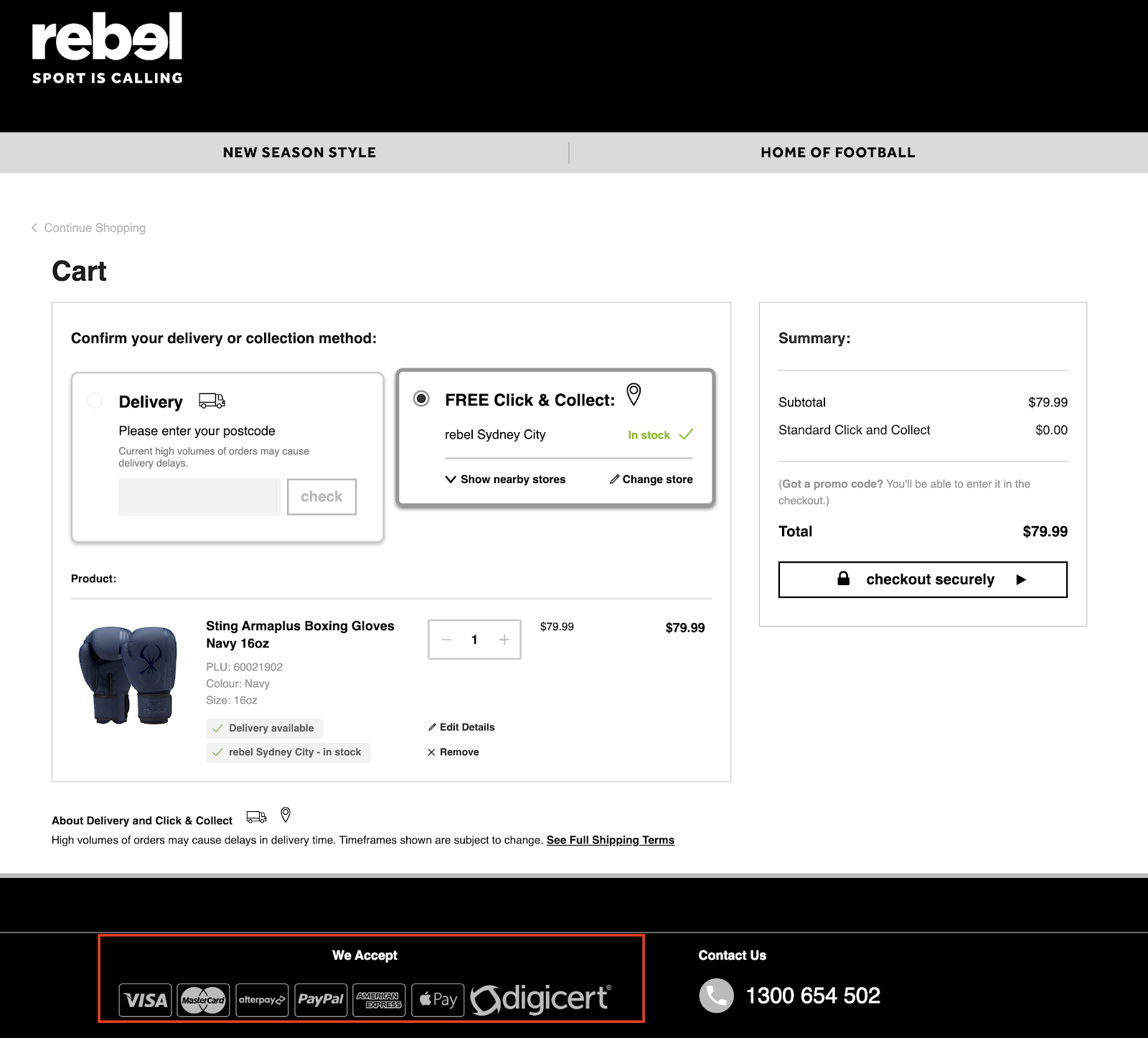This is a detailed screenshot of the Rebel website. In the top left corner, the website's name, "Rebel," is displayed with the second 'E' written backwards. The top section has a black background with the website name in white text. Below this, there are two prominent gray rectangles. One reads "New Season Style," while the other states "Home of Football."

A button labeled "Continue Shopping" is presented in a smaller font below these rectangles. In larger font, "Cart" is displayed prominently. The main box on the screen prompts users to confirm their delivery or collection method and highlights "Delivery or Free Click and Collect," with "Rebel Sydney City In Stock" being the selected option.

The product listed is a pair of Sting Arma Plus Boxing Gloves in Navy, weighing 16 oz, priced at $79.99. To the right, there's a summary of the order showing a subtotal and total of $79.99 each, along with a "Check Out Securely" button.

At the bottom left, the website features accepted payment methods, including Visa, MasterCard, Afterpay, PayPal, American Express, Apple Pay, or DigiCert, within a rectangle with a red border. To the right of this section, there's a "Contact Us" option, featuring a contact number: 1300-654-502.